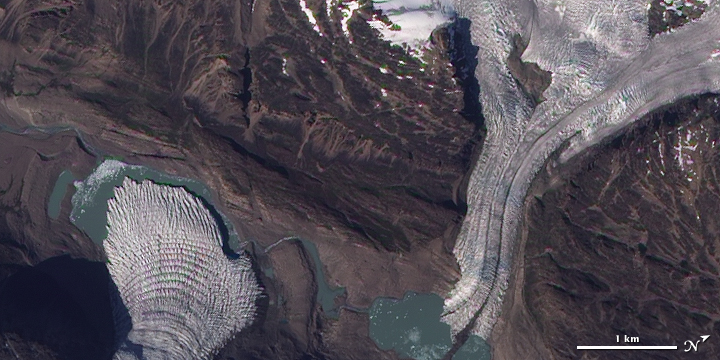This aerial photograph captures a stunning landscape featuring glaciers, ice sheets, and a mix of rugged hills and mountains. Dominating the scene are undulating hills in various shades of dark and light brown, with a notable light brown, flat band extending from the lower left. The image also includes green-colored bodies of water, highlighted by a striated white ice sheet in the lower left that merges seamlessly into these water bodies. On the right side of the photograph, a dramatic river of ice cascades down the mountainside into a larger body of water. Scattered across the upper left and center areas are patches of white, likely snow. In the lower right corner, a scale indicating "one kilometer" is visible along with an 'N' and an arrow pointing to the upper right, suggesting the direction of north. The intricate details vividly encapsulate the dynamic interaction between the ice and the surrounding terrain.